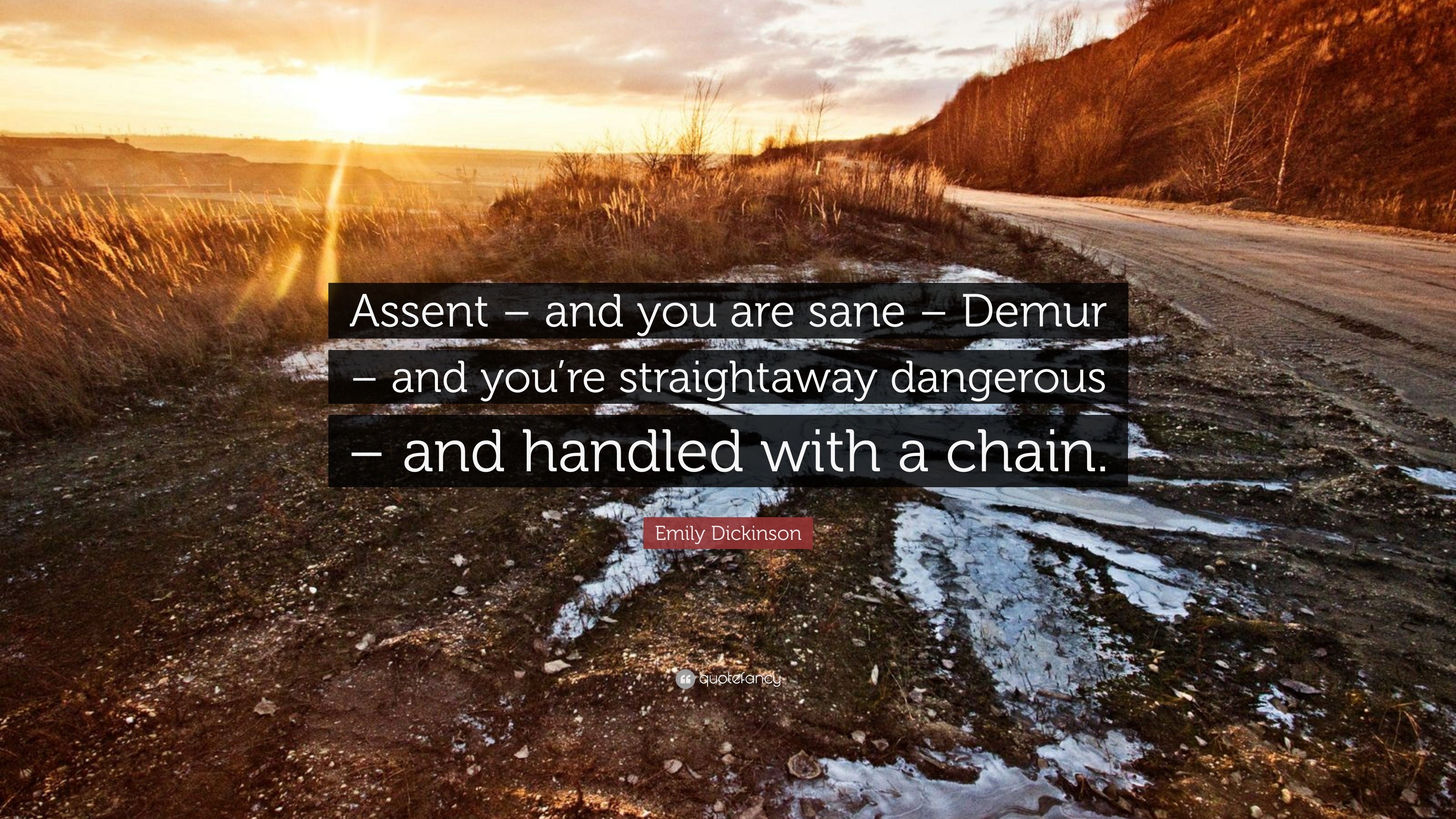This rectangular outdoor photograph, approximately 6 inches wide and 3 inches tall, captures a serene yet poignant scene during the daytime. Dominating the upper right-hand corner is a small hillside that slopes gently downwards towards the left, leading to a paved road that traverses the image from halfway down the right-hand side and extends across to the left. The road narrows as it meets the edge of the hill, where remnants of snow and ice linger within the old tire tracks of the roadside gravel or dirt.

In the distance on the left, fields of wheat or tall grass sway gently, set against the backdrop of a yellow-orange setting sun that bathes the entire image in a warm, golden-brown hue. This sun sits atop the skyline, offering a scenic view of valleys below and casting a nostalgic amber glow over the landscape.

Central to the image are three semi-transparent black rectangles with white text, which read in sequence: "Ascent, and you are sane, demure," "— and you are straightaway dangerous," "— and handled with a chain." These poignant lines are followed by a red background with white text attributing the quote to Emily Dickinson. This blend of natural beauty and profound literary reference imbues the photograph with a contemplative and evocative atmosphere.